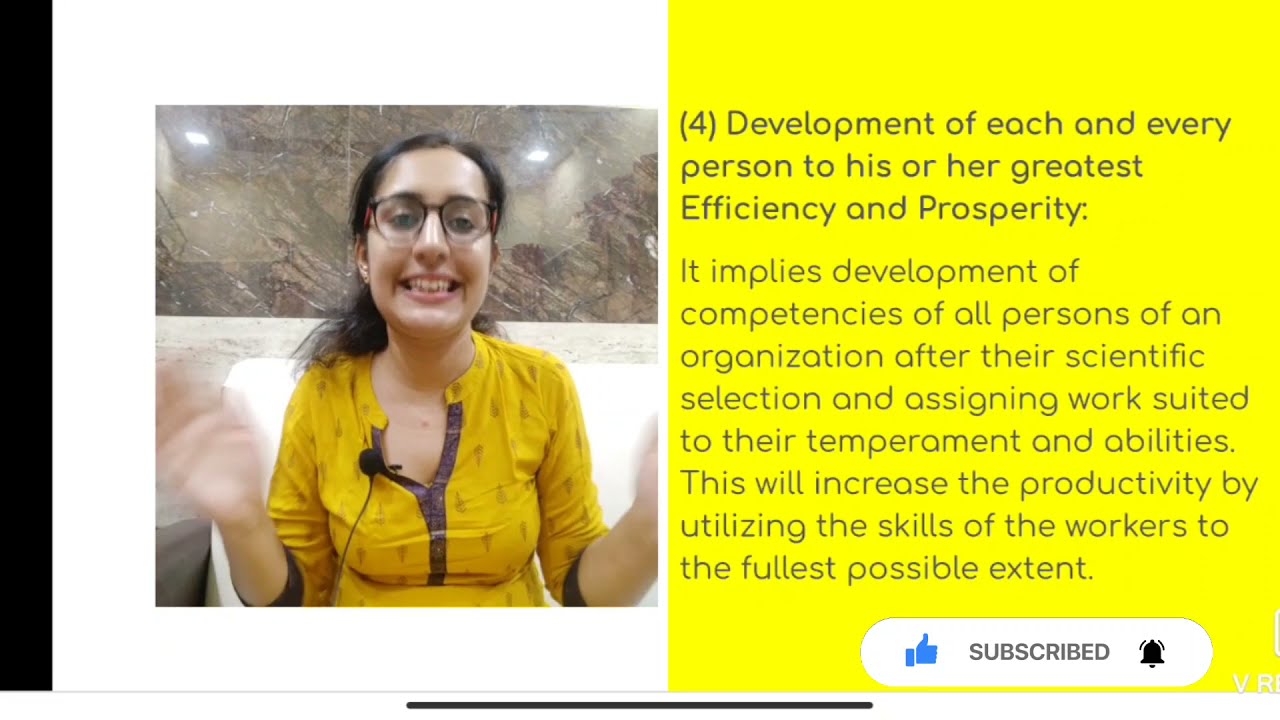The image is a photograph of a young woman in her late 20s, wearing glasses and smiling warmly. She has long dark hair and is dressed in a golden yellow blouse with brown fringes and patterns. A microphone is attached to her blouse, which droops slightly where the microphone hangs. She's seated in front of a marble-looking wall and appears to be enthusiastically gesturing with her hands, which are blurred due to her rapid movements. To the right of her is a long piece of text labeled as "Number 4," discussing the development of each individual's efficiency and prosperity within an organization by scientifically selecting and assigning tasks that suit their temperament and abilities. This maximizes productivity by fully utilizing the workers' skills. At the bottom of the text, there are icons for thumbs up, subscribe, and a bell notification.